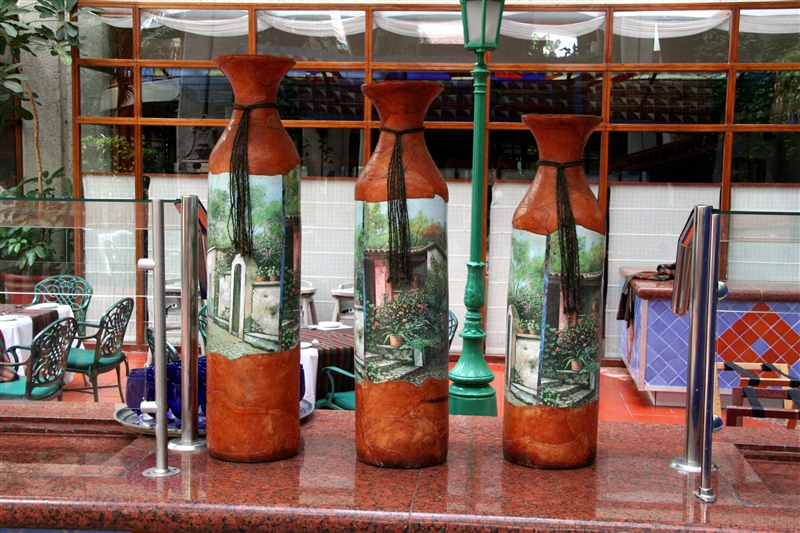The image captures three tall, decorative clay vases arranged in descending height from left to right on a reddish granite countertop, possibly in an outdoor restaurant setting. Each vase displays a segment of an identical painting depicting a bucolic scene with a stone fence, an archway, trees, a brown house, and flowers, perfectly capturing the establishment’s aesthetic. The vases sport a reddish-brown pottery hue and are adorned with tassels or cords tied around their necks just below where they flare out. Background elements include a white brick wall, several tables and chairs, and another counter, suggesting the likely placement of the containers within a bar or dining area surrounded by expansive windows that let in ample natural light.